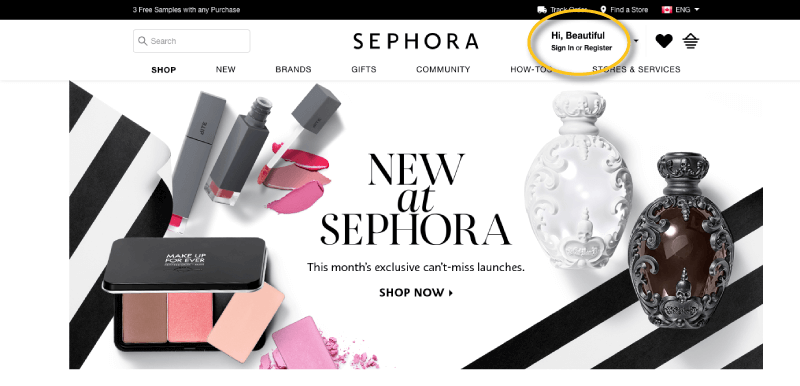Screenshot of a Sephora webpage: At the top, a black navigation bar runs across the page, adorned with white text on the left. On the right side of the bar, there are options to "Track Order," "Find a Store," and select a "Language." Below this, the header prominently displays the Sephora logo, with a centered search bar to the left and icons for a shopping cart and favorites list to the right. Additionally, there is a greeting that reads "Hi, Beautiful—Sign In or Register," highlighted by a yellow outline circle. 

Beneath the header, a navigation menu offers various options such as "Shop," "New," "Brands," "Gifts," "Community," "How-To," and "Stores & Services." The main body of the webpage features an elegant composition of beauty products, including lipstick and perfume, set against a mostly white background with black and white lines decorating the corners and left side. Centrally, bold text announces "New at Sephora: This month, exclusive can't-miss launches. Shop now." Prominently displayed to the left are two perfume bottles, one white and the other black.